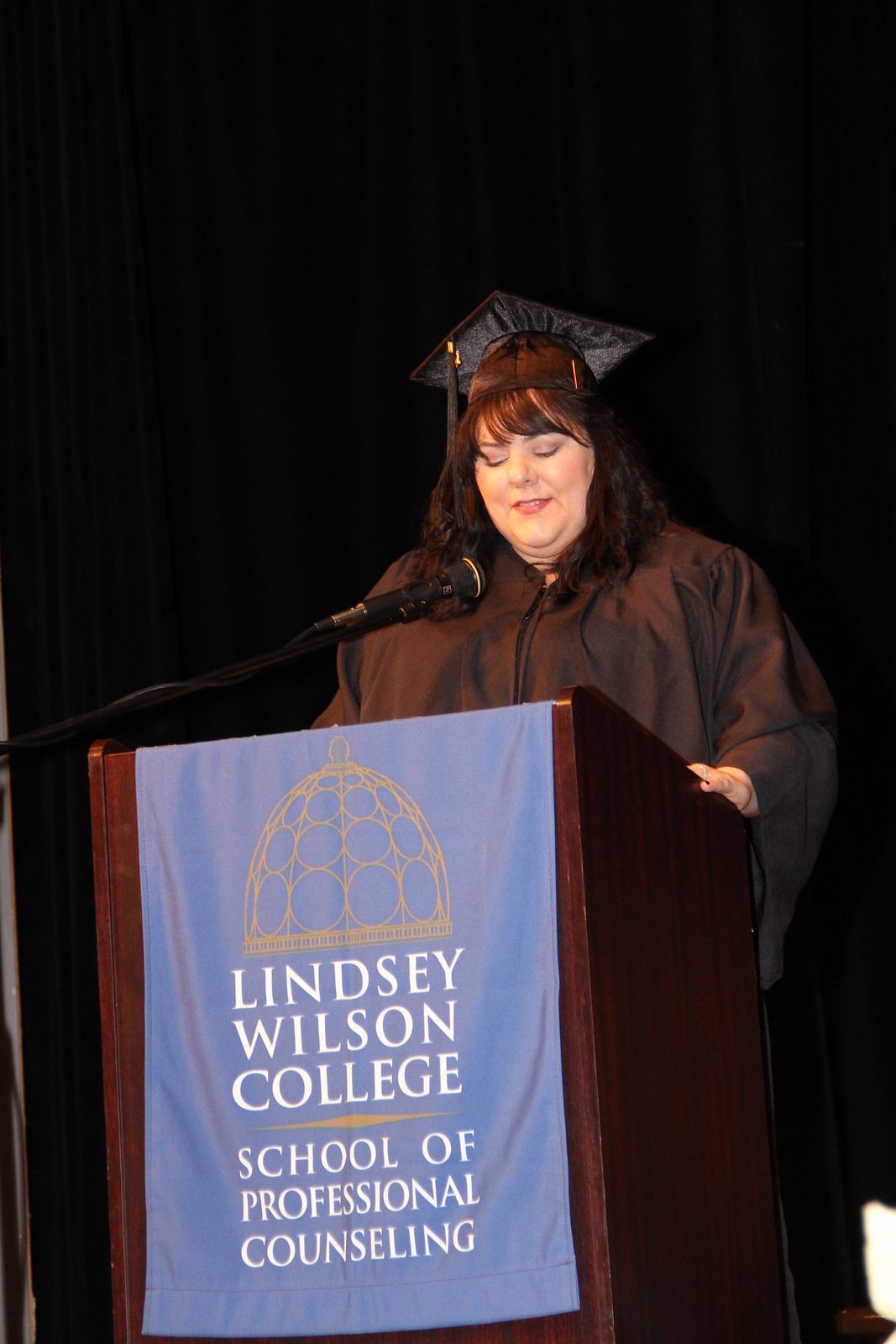In this detailed photograph, a woman, possibly a graduate, stands at a podium delivering a speech during what appears to be a graduation ceremony. The setting is indoors, characterized by a very dark black background. She wears a traditional black cap and gown, her dark brown hair visible underneath the cap, and she appears to have bangs. Her left hand rests on the podium while she looks downward, her eyes seemingly closed, indicating a moment of reflection or focus.

The podium prominently displays a blue sign with a gold graphic of a building, possibly a cupola, and bears the text "Lindsay Wilson College School of Professional Counseling." The setting is dimly lit but a spotlight intensely illuminates her, casting light predominantly on her and creating a stark contrast with the somber backdrop. In the bottom right-hand corner, a flash of light adds to the atmospheric ambiance of the scene.